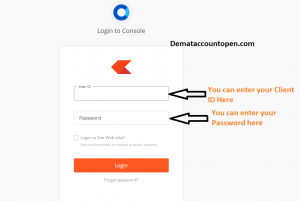This is a detailed screenshot of a login interface on a mobile application or a cell phone screen. The interface is housed within a light gray, rectangular box, which is oriented in landscape mode. 

At the top of the interface, there is a blue circle with a gray center matching the background. The circle is predominantly dark blue, transitioning to a lighter blue on the right quarter. Inside the circle, in black text, it says "Login to Console." Adjacent to this circle, the text "DematAccountOpen.com" is prominently displayed.

Below this header, there is a white, credit card-sized box positioned in portrait mode. The top of this box features an orange arrow pointing left. Beneath the arrow, there is a field labeled for entering the client ID. Below this, there is another field designated for entering the password. Adjacent to this password field is a checkbox with some unreadable text next to it. At the bottom of the white box, there's a large orange button labeled "Login."

On the right-hand side of the interface, there is a black arrow pointing towards the client ID field, accompanied by an orange instruction: "Enter your client ID here." Similarly, another black arrow points towards the password field, with an orange instruction: "Enter your password here."

The overall design is clean and instructive, guiding the user step-by-step through the login process.